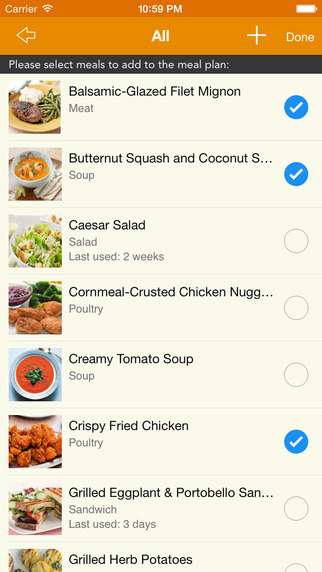A smartphone screen displays a meal planning app with an orange header. At the top, the status bar features a white "carrier" label, a volume icon, the time "10:59 PM," and a fully-charged battery icon. Below, a lighter orange bar includes a left-pointing arrow, the word "All" in the center, and a "Done" button, all in white.

The main section of the screen features a white background with a prompt that reads, "Please select meals to add to the meal plan..." in black text. The following meal options are listed:

1. **Balsamic Glazed Filet Mignon** (Meat):
   - Image: Filet mignon served with green beans and potatoes on a yellow plate.
   - Status: Selected (indicated by a blue box with a white check mark).

2. **Butternut Squash and Coconut Soup** (Soup):
   - Image: A white bowl filled with orange-colored soup.
   - Status: Selected (indicated by a blue circle with a white check mark).

3. **Caesar Salad** (Salad):
   - Image: A large bowl of Caesar salad.
   - Note: "Last used two weeks ago."
   - Status: Not selected (indicated by a gray box).

4. **Cornmeal Crusted Chicken Nuggets** (Poultry):
   - Image: Large chunks of browned chicken nuggets served with broccoli and a purple vegetable in a bowl.
   - Status: Not selected.

5. **Creamy Tomato Soup** (Soup):
   - Image: A large white bowl filled with tomato soup.
   - Status: Not selected.

6. **Crispy Fried Chicken** (Poultry):
   - Image: A large plate of crispy, browned fried chicken.
   - Status: Selected (indicated by a blue circle with a white check mark).

7. **Grilled Eggplant and Portobello Sandwich** (Sandwich):
   - Image: A sandwich made with grilled eggplant and portobello mushrooms on toasted bread.
   - Note: "Last used three days ago."
   - Status: Not selected.

8. **Grilled Herb Potatoes** (partially visible):
   - Image: Double-baked grilled herb potatoes.
   - Status: Not selected. 

The descriptions and selection statuses provide a user-friendly interface for efficiently planning meals.